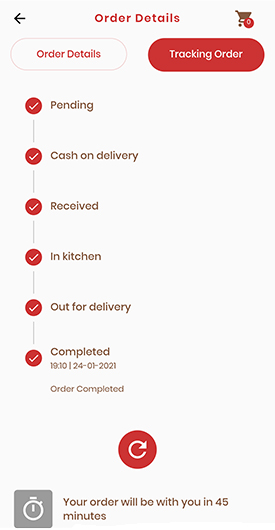A detailed screenshot of an order menu is depicted with a light gray background forming a tall rectangular frame. At the very top left corner, a left-pointing arrow is situated, followed by the text "Order Details" in red font. On the top right, a small shopping cart icon displays zero items.

Beneath this header, two buttons are visible: "Order Details" and "Tracking Order." The "Tracking Order" button is active, indicated by its red background.

Below the buttons, a list of order statuses is displayed, each marked with a red circle containing a white checkmark. The statuses are: Pending, Cash on Delivery, Received, In Kitchen, Out for Delivery, and Completed. The status of "Completed" is followed by the date "24-01-2021" and the text "Order Completed."

A circular refresh button is located below the statuses. At the bottom of the menu, a clock icon in a gray box appears on the left, accompanied by the text "Your order will be with you in 45 minutes" on the right.

This screenshot likely represents a tracking interface for a delivery order.